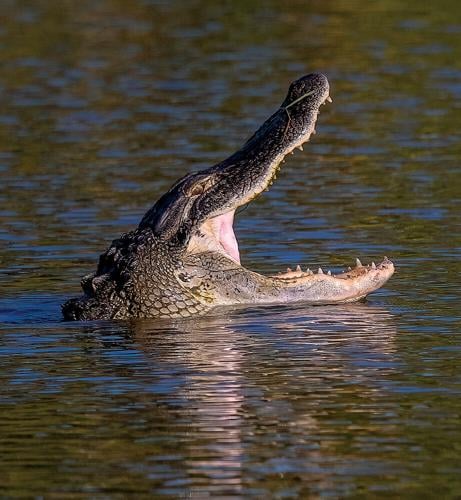In this striking image, a large alligator floats in the middle of murky, dark green-gray water that might be part of a swamp. The scene is bathed in mid-evening daylight, with sunlight reflecting off the water’s surface, suggesting a clear blue sky above. The water has some small wave action, adding texture to the otherwise still scene.

The alligator commands attention as it faces the right side of the image, its mouth wide open at an impressive 45-degree angle, almost appearing to yawn. Its fearsome array of pointy teeth is fully visible above and below its large jaw. There is a hint of pink at the hinge of its jaw, contrasting with its predominantly gray color. The scales on its head are substantial and irregular in shape, with a tinge of green accentuating its jawline and chin.

Its eyes, which are very tiny, appear closed or possibly impaired, adding to the enigmatic aura of the creature. The robust, scaly texture of its back features visible knobs, emphasizing its formidable presence. The murky water with its mix of brown and green hues and slight wave action enhances the wild, untamed feel of the scene, capturing a moment of natural intensity and raw beauty.